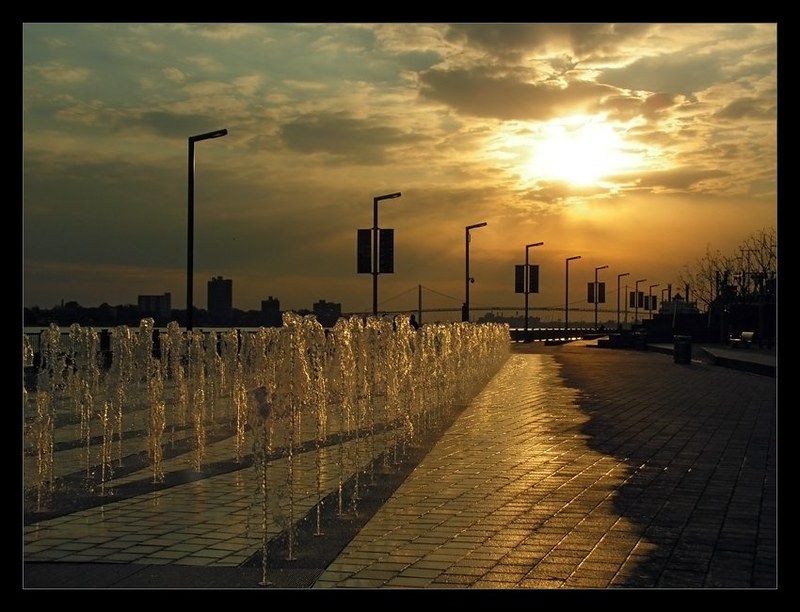The photo captures a picturesque urban scene just before sunset. The focal point is a series of miniature cooling fountains embedded in a brick walkway, positioned beside a serene river. The water jets, spaced at regular intervals, shoot up about a foot or two into the air, creating a mesmerizing effect as the droplets glisten in the diminishing light. The surrounding walkway has acquired a reflective sheen from the water splashes. To the left, the city skyline stands silhouetted against the evening sky, with cloud cover enhancing the dramatic ambiance. Streetlights and possibly parking meters remain unlit along the distant backdrop, adding to the quiet, almost suspended quality of the scene. The overall composition suggests a tranquil coastal view, harmoniously blending elements of natural beauty and urban architecture.